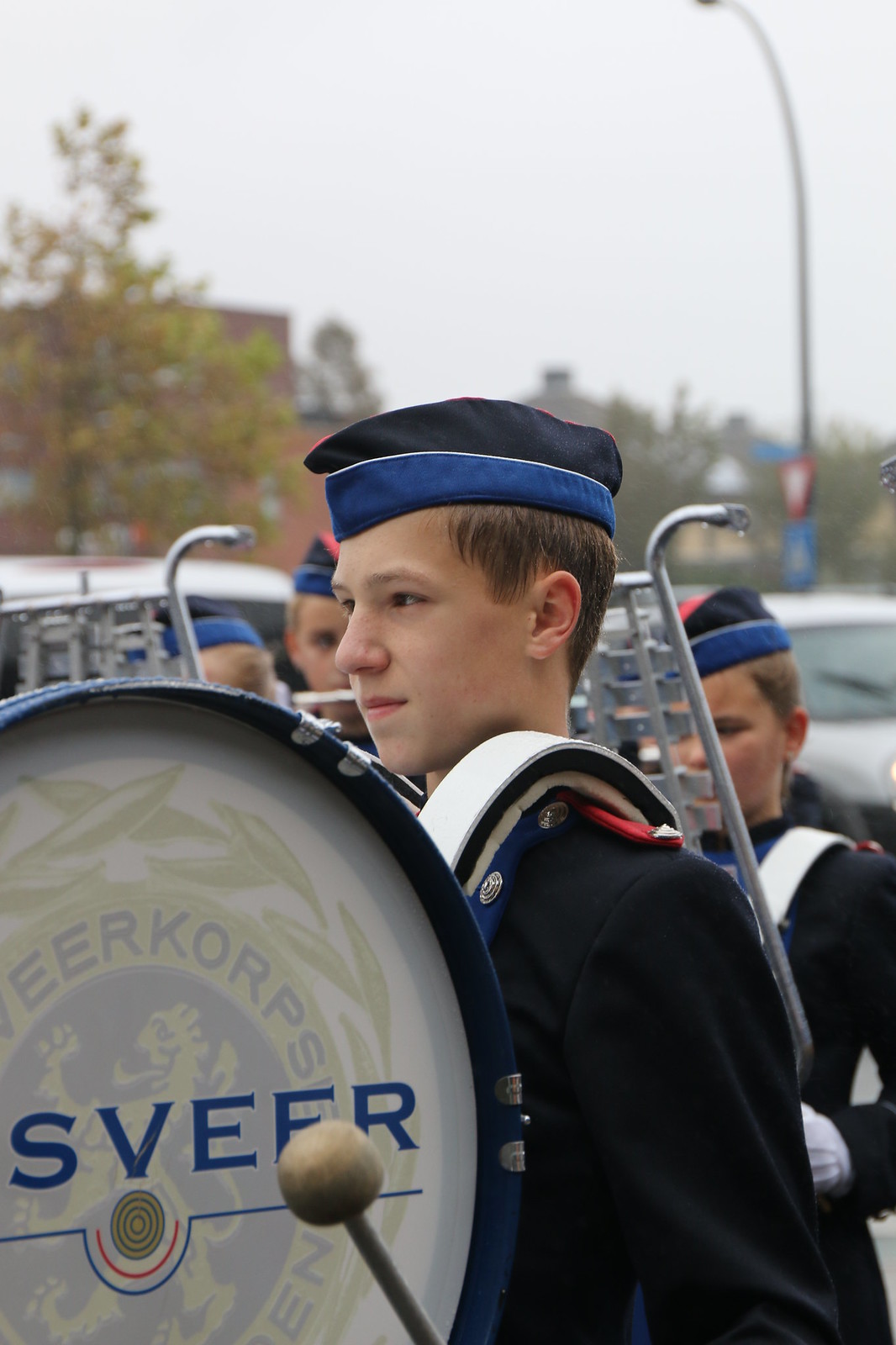The image captures a lively scene of a marching band comprised of boys and girls dressed in crisp, matching uniforms. At the front and center is a young boy, his drum set securely strapped to his upper body. He is caught in a moment of concentration, glancing to the left of the image. Adorning his head is a sharply styled hat that completes his band attire. 

Behind him, his fellow bandmates, also in full uniform and hats, are arranged in formation, each carrying their respective instruments. While the figures at the back are blurry, they contribute to the sense of depth and motion in the photograph. 

In the distance, various elements of the surroundings come into view—a few vehicles, a tall building, and an array of trees enrich the backdrop. Overhead, the clear sky adds a touch of brightness, enhancing the overall vividness of the scene. It's evident that the picture was taken in natural light, contributing to the sharp focus on the boy and his drum at the forefront while softly blurring the detailed background.